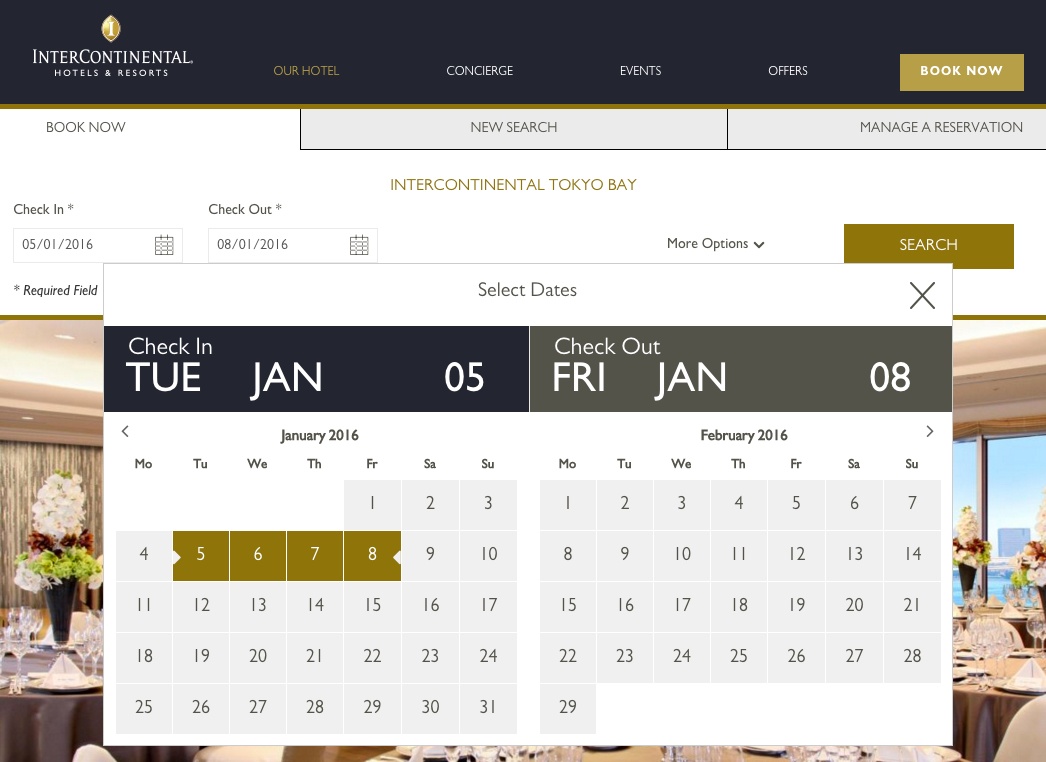The interface for booking at the Intercontinental Hotel and Resorts is detailed and user-friendly. At the top, the page is branded with the "Intercontinental Hotel and Resorts" name prominently displayed on the navigation bar. The bar includes options for "Our Hotel," "Concierge," "Events," "Offers," and a distinct gold button with white font labeled "Book Now."

Below the navigation bar, a gold line separates the menu from the booking options. To the left, there is a "Book Now" link, the center displays "New Search," and to the right, there's a "Manage a Reservation" link. Beneath these options, in the center, "Intercontinental Tokyo Bay" is written in gold.

On the left side of the main booking section, users can input their check-in and check-out dates. The current check-in date entered is January 5, 2016, while the check-out date is August 1, 2016. Each date field has an accompanying calendar icon for easy selection. To the right, there's a "More Options" dropdown and a gold "Search" button to proceed with the booking.

A popup calendar interface shows up when selecting dates. For check-in, the calendar highlights Tuesday, January 5, 2016, and includes selectable dates from January 5 to January 8. However, for the check-out field, Friday, January 8, 2016, no dates are highlighted, suggesting a possible error since the check-in and check-out dates span an unusual three-month period.

This detailed user interface ensures easy navigation and booking for guests at the Intercontinental Tokyo Bay, despite the noted anomaly with the date selection.